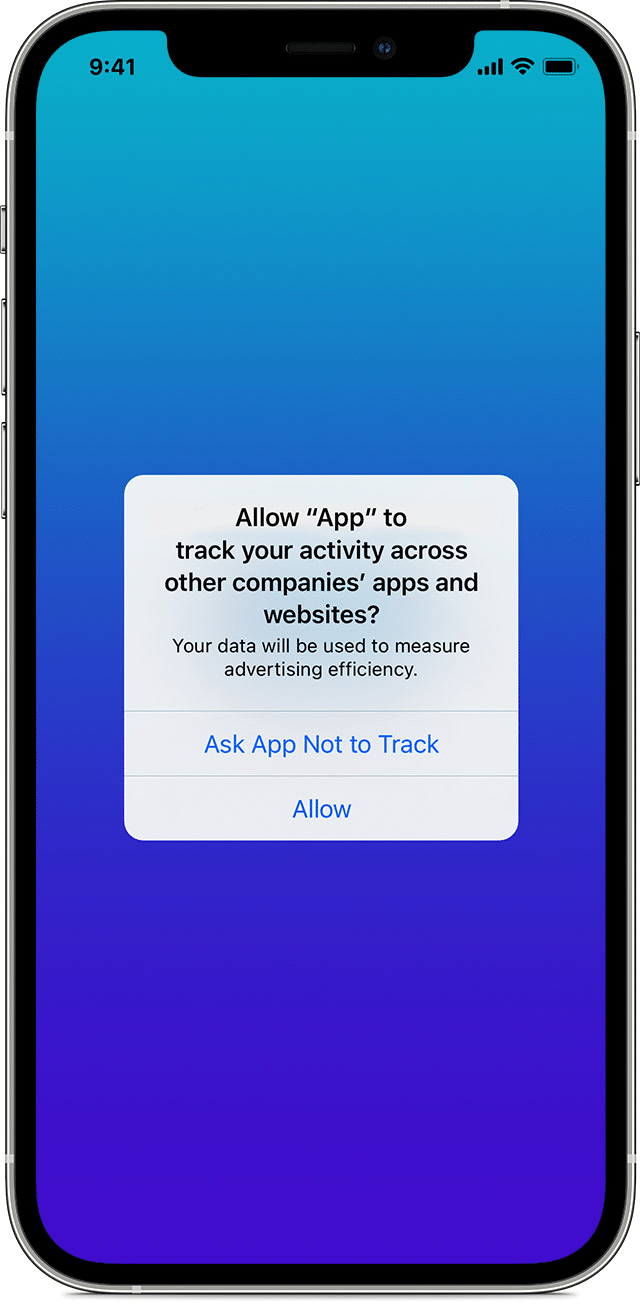A smartphone screen displays an app notification with the message: "Allow App to Track Your Activity Across Other Companies' Apps and Websites? Your data will be used to measure advertising efficiency." Options are given to either "Ask App Not to Track" or "Allow." The screen shows it is 9:41 AM in the top left corner, with full bars of data, Wi-Fi signal, and a fully charged battery. The background is a gradient blue screen, starting off lighter at the top and gradually getting darker towards the bottom. The phone's power button is visible on the right side, while the volume buttons are on the left. The top of the phone features a speaker and a camera.